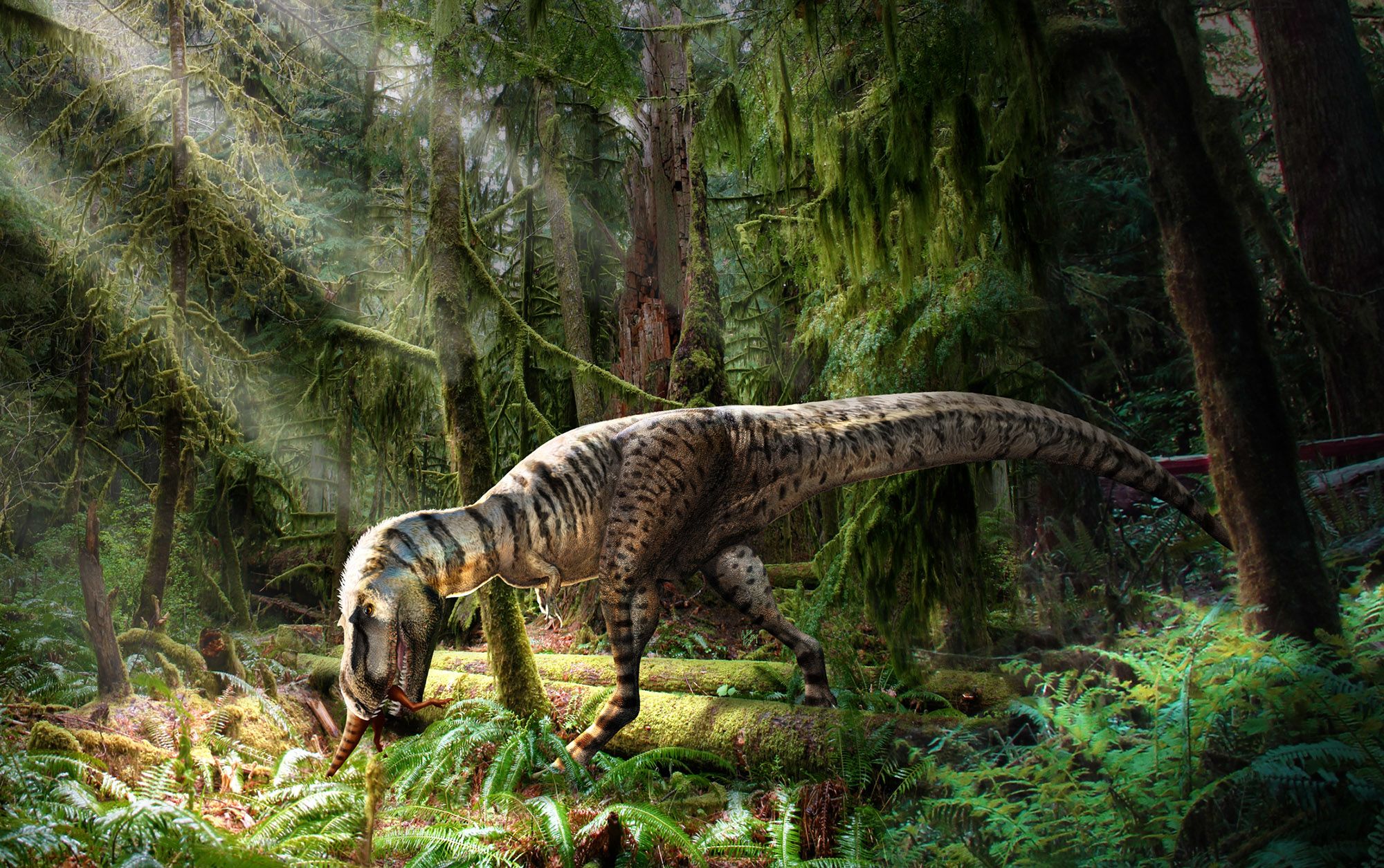The image depicts a vibrant, detailed scene in a dense, prehistoric forest, likely AI-generated. At the center is a large, gray T-Rex with black stripes and polka dots, standing triumphantly amid a lush, rainforest-like environment brimming with towering trees, fallen logs covered in moss, and an abundance of ferns and foliage. The T-Rex, characterized by its small arms and powerful legs, is in the midst of consuming a smaller dinosaur, with only bright red legs and an orange and black striped tail visible protruding from its mouth. The ambiance is further enriched by the sunlight piercing through the dense canopy, casting a warm, radiant glow from the top left corner, enhancing the scene's vibrant and humid atmosphere. The entire setting evokes a sense of raw, primitive nature, devoid of any modern civilization, showcasing an era where dinosaurs reigned supreme.